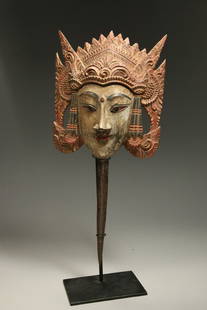In this vertically oriented, realistic photograph, an ancient-looking mask sits prominently on a tall, black metal stand adorned with a square base. The background features a dark upper section transitioning into a white lower section, which contrasts sharply with the mask. The mask itself, most likely made of wood or a hard composite, exudes an aura of antiquity and cultural significance. It depicts a yellow-tan face with a serene, stoic smile, characterized by large sweeping eyebrows, almond-shaped eyes, and a long nose. A red dot accentuates the center of its forehead, possibly hinting at Indian origins.

The most striking feature of the mask is its ornate, red crown that extends both upwards and downwards, forming a protective square frame around the face. The crown is detailed with red spikes, including two prominent ones on each side that taper down towards the chin. The mask appears lifelike with its pointed chin and meticulously sculpted features, including deeply set dark eyebrows, vivid red lips, and almond-shaped eyes that suggest an ancient, yet timeless, visage.

While the mask's complexion is lighter with hues of brown and tan, its crown echoes a reddish, almost rust-colored hue, adding to its regal appearance. The cylindrical pole of the stand, subtle yet sturdy, melds into the base, providing an elegant support for this exquisite piece. This photograph captures not just an artifact, but a slice of ancient artistry, possibly intended for display in a museum or as a unique piece of home décor.